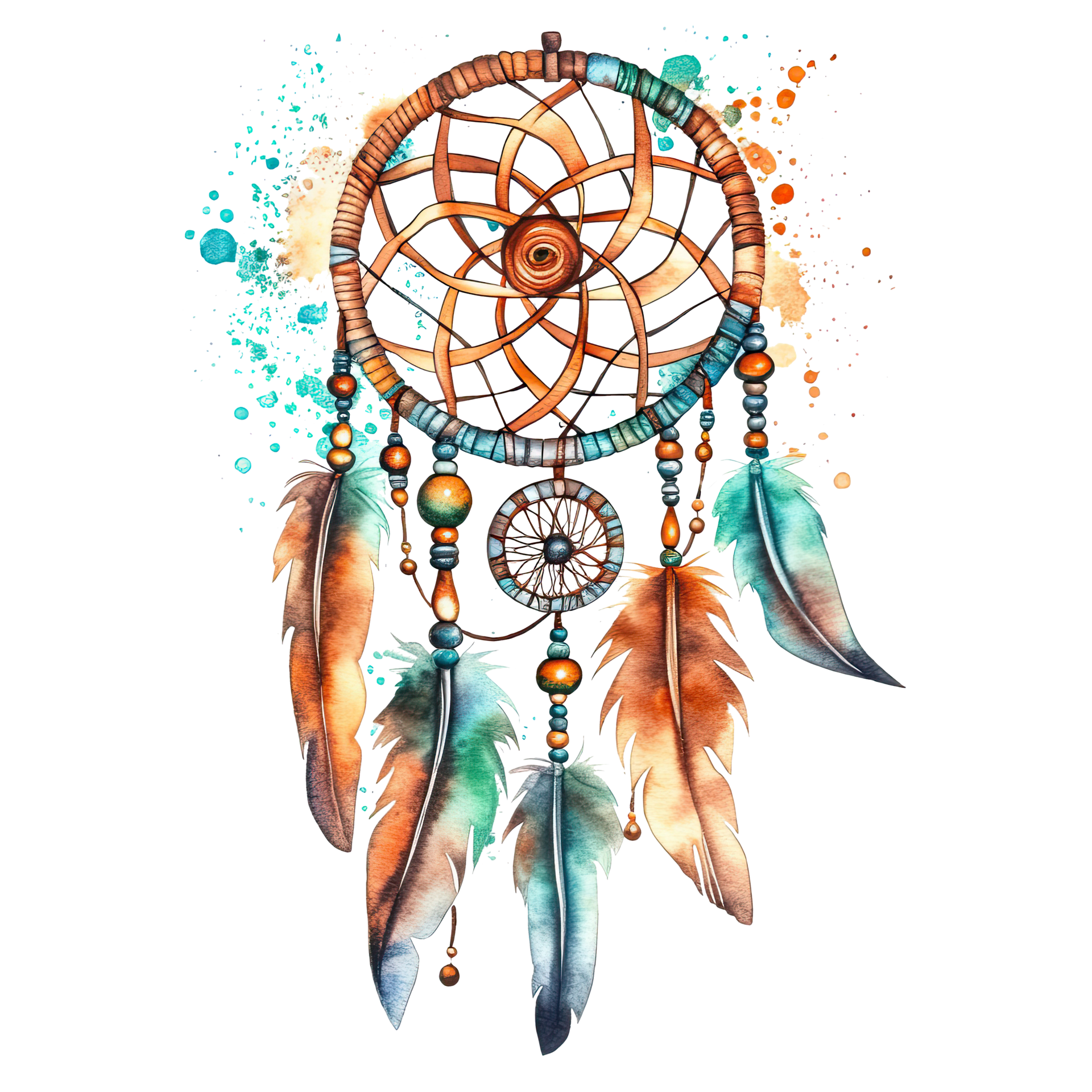This image showcases a watercolor painting of a dreamcatcher against a white background, adorned with delicate ink splotches and dots that span from light turquoise blue on the left to vibrant shades of orange and red on the right. The dreamcatcher features a circular outer edge entwined with a wire, blending colors of brown, orange, blue, and turquoise. The center displays an intricate web design resembling a flower pattern, created with strings in varying shades of brown and tan. Five feathers, extending from the base, are decorated with beads and embrace a palette of orange, blue, turquoise, yellow, and tan, harmonizing with the dreamcatcher's overall aesthetic. The splattered paint adds an artistic touch, enhancing the ethereal beauty of this illustrated dreamcatcher.